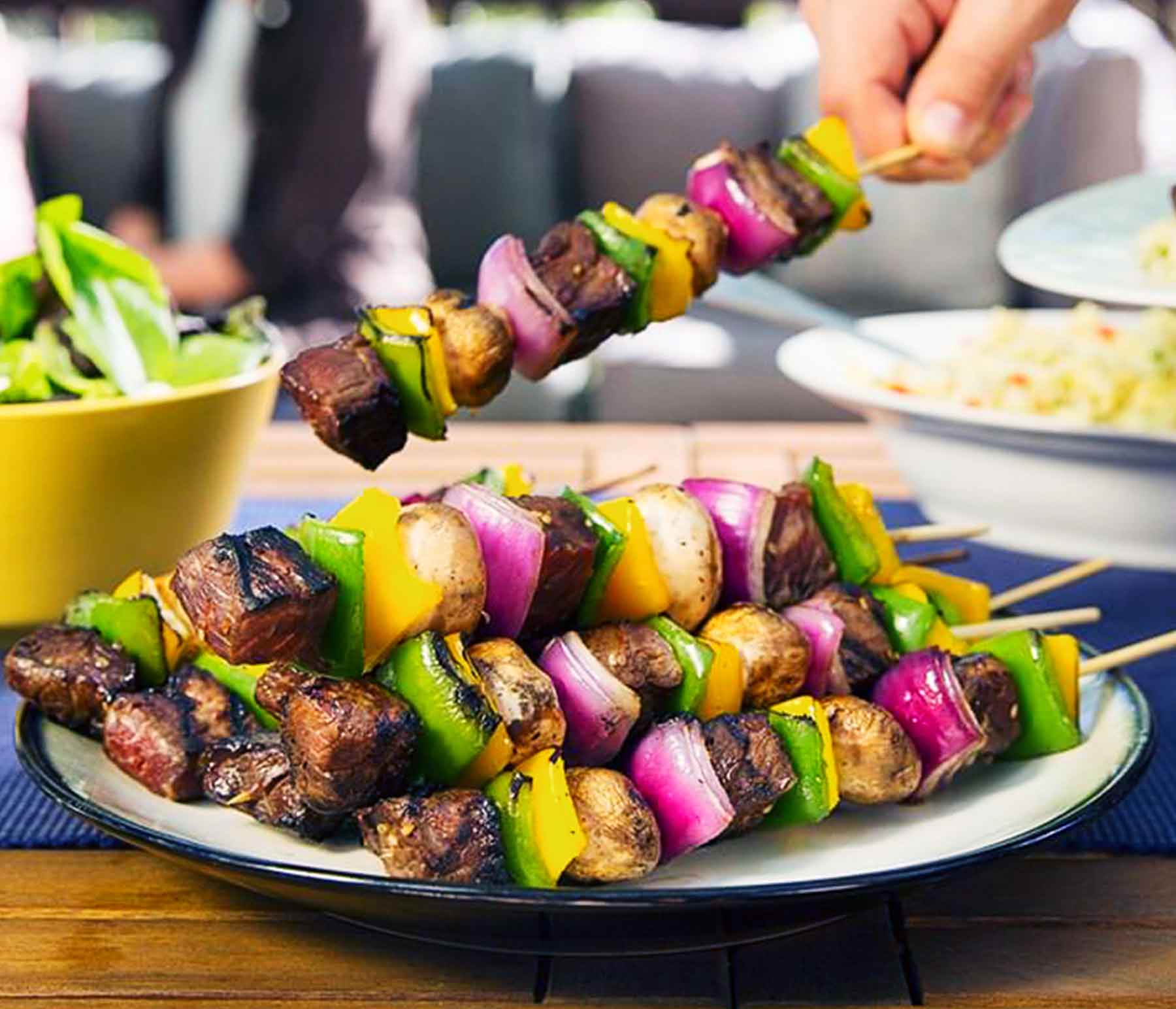This is a color photograph in landscape orientation, capturing a vibrant tabletop scene centered on a round white platter with a dark blue rim, piled high with about eight steak kebabs. The kebabs are artfully arranged, featuring sections of brown, grill-marked steak interspersed with colorful vegetables—green and yellow bell peppers, red onion wedges, and mushrooms—all threaded on wooden skewers. Positioned on a brown wood table with a blue mat partially underneath, the scene is accented by a person's hand emerging from the upper right corner, grasping one of the kebabs. To the left of the platter is a yellow bowl filled with fresh green salad, while on the top right, there is a white bowl containing rice with a spoon. The background is softly blurred, hinting at other diners without distracting from the vividly detailed food in the foreground.